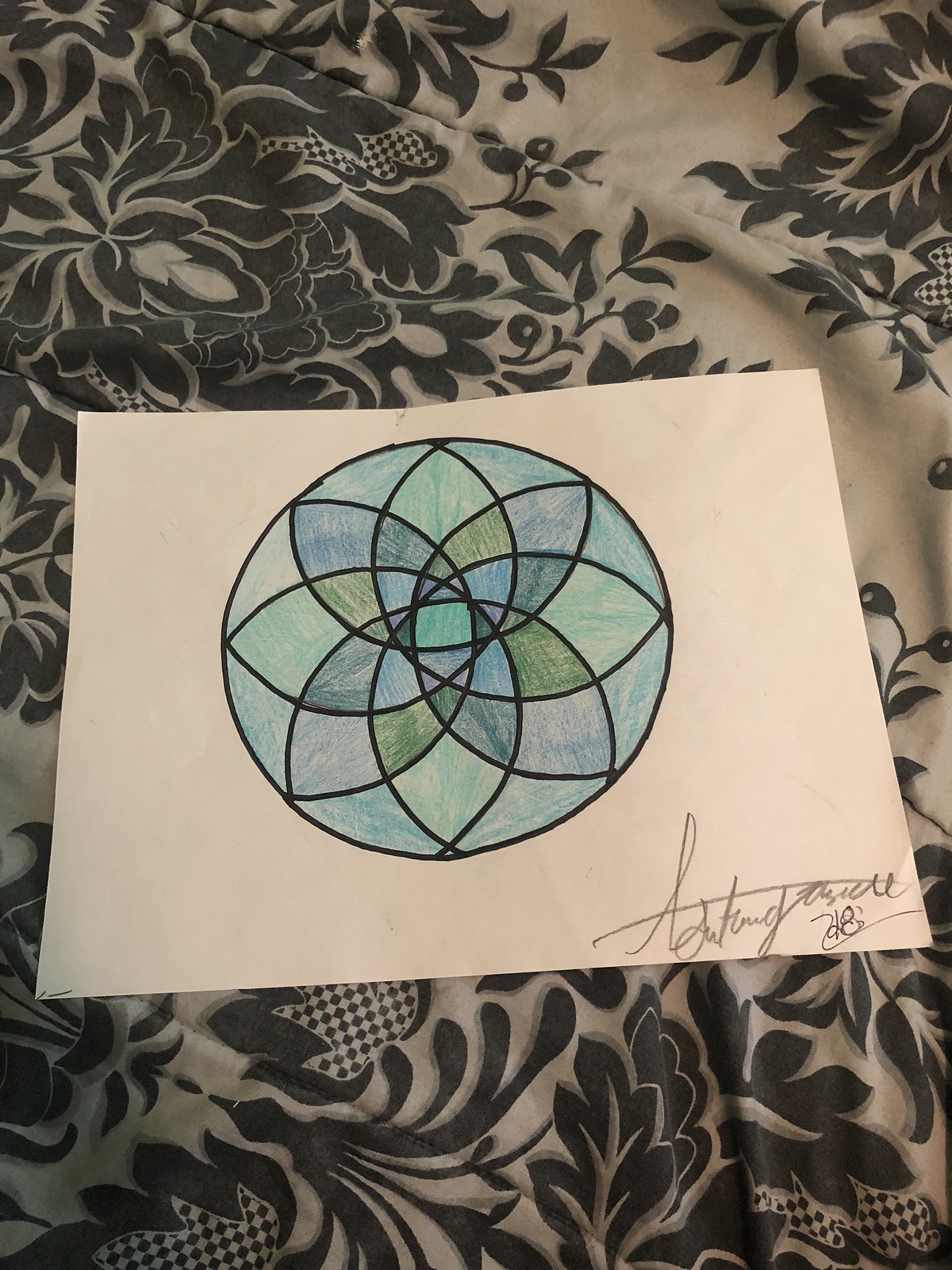The image features a meticulously detailed drawing on a white piece of paper, which is placed atop a white and black floral-patterned tablecloth or curtain. The artwork depicts a complex, abstract floral pattern, consisting of a large black-outlined circle at its center. Within this circle, smaller overlapping spiral circles create a mesmerizing mosaic of vibrant colors, including various shades of blue, teal, green, purple, brown, and olive. The overlapping circles intersect to form distinct sections, each filled with different hues, giving the piece a rich and textured appearance. At the very center of the design, there is a prominent teal square. The intricate lines and colors appear to be drawn with different art pencils, enhancing the depth and structure of the piece. In the bottom right-hand corner of the paper, the artist has signed their name in cursive with a light gray pencil, accompanied by an indecipherable date, which includes an eight. Despite the signature being somewhat unreadable, it adds a personal touch to the stunning and vibrant composition.